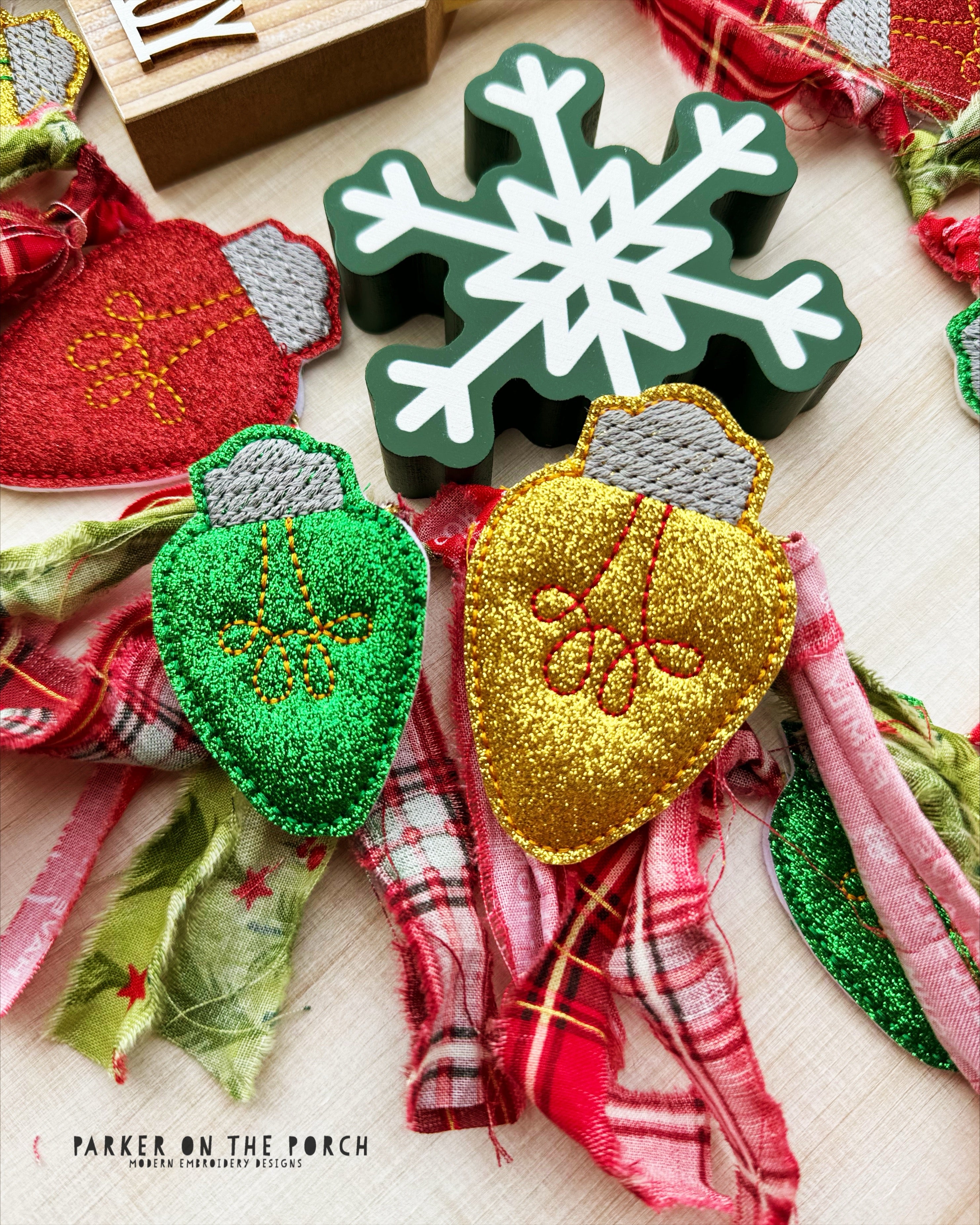This advertisement from Parker on the Porch, highlighted by a watermark in black lettering in the lower left corner, showcases a vibrant collection of modern embroidery designs arranged on a pale wooden surface. Central to the image are intricately detailed Christmas-themed embroidered fabric patches—representing festive Christmas lights—with three prominent pieces: a red, a green, and a gold light, each featuring glittery, sparkly fabric with thread embroidery detailing the spiral light coil. Accompanying these are fabric strips with frayed edges in various Christmas colors and designs, adding depth and texture to the display. At the upper portion of the image, a green cutout featuring a white snowflake motif can be seen, alongside the partial edge of a wooden block-shaped craft. Together, these elements craft a vivid, festive scene intended to inspire and showcase Parker on the Porch's sophisticated embroidery creations.